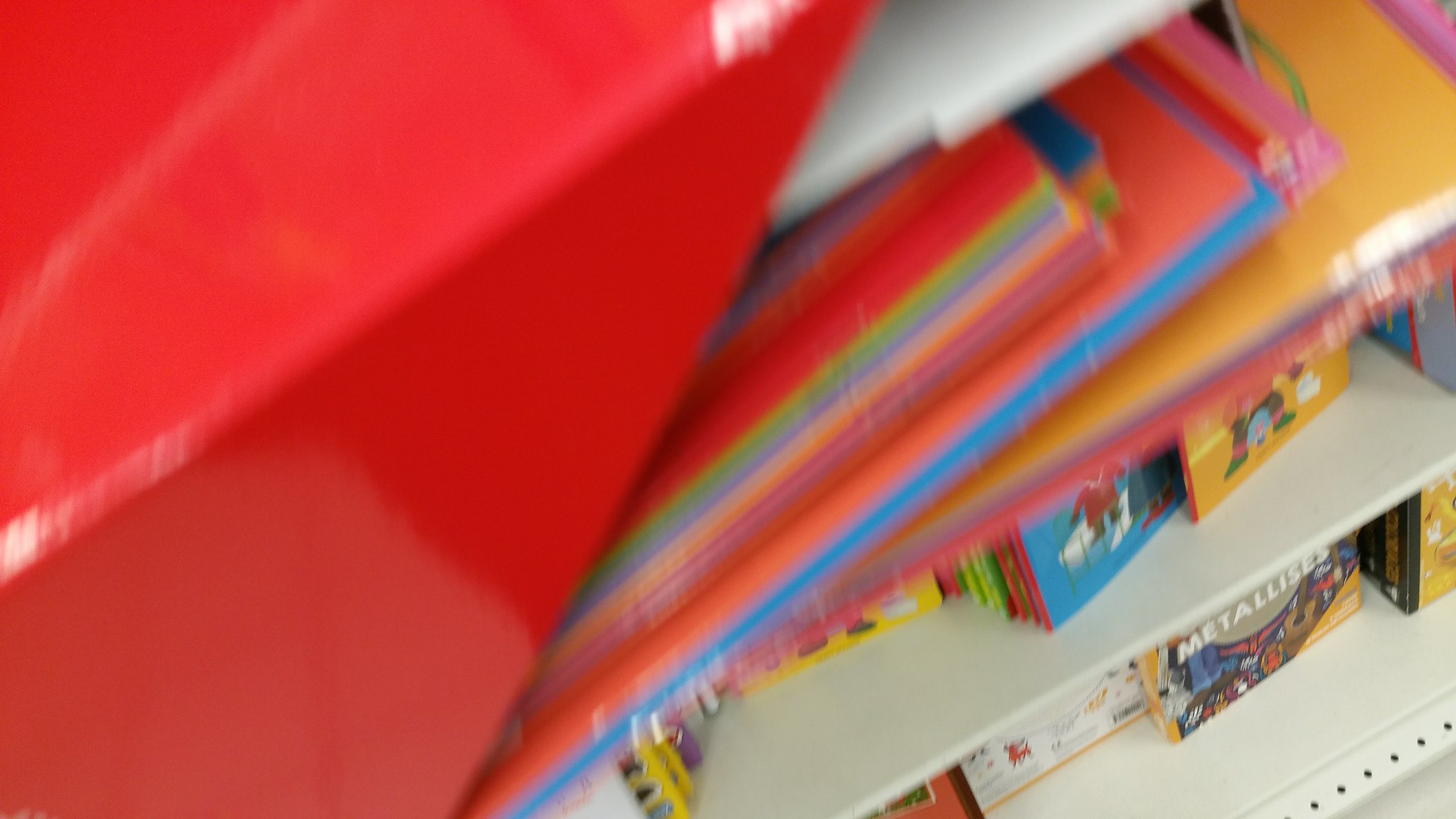This image captures a detailed top view of a multi-tier metal bookshelf. The bottommost shelf features a unique notebook paper-like design with corrugated edges and multiple small holes. This shelf houses several items, possibly books or games, with one clearly labeled "Metallesis." 

The second shelf from the bottom contains an array of colorful books. Although only the bottom portions of the books are visible, their spines display vibrant hues of red, blue, and orange, adorned with images of people, granting the shelf an eclectic and lively appearance.

The top shelf is filled with a stack of construction paper, showcasing a full spectrum of rainbow colors, adding a burst of visual delight and completing the visually engaging composition of the bookshelf.